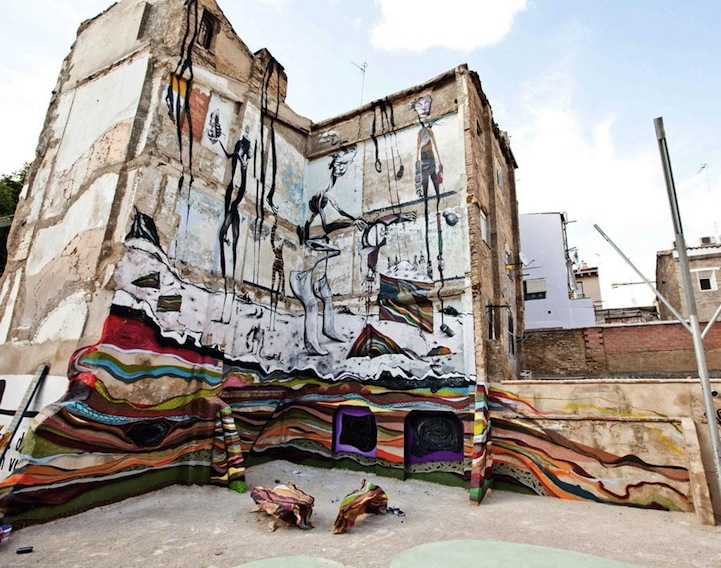The image depicts an old, vintage stone building, likely situated in a foreign country, surrounded by other buildings visible in the distant background. The building’s façade features intricate graffiti, which predominantly covers its lower portion and creates a striking visual effect with layers of wavy, multicolored stripes—greens, purples, oranges, yellows, and blues—reminiscent of sedimentary layers. This base of vibrant colors gives way to detailed, surrealist depictions of long, slender people, painted above in more muted monochromatic tones of beige, black, and white. Some parts of the graffiti give the impression that the building is melting. Adjacent to this building is a wall that also carries graffiti, creating a seamless extension of the artwork. The scene is set against a backdrop of a light blue sky with scattered white clouds, and there is a glimpse of a tree on the far left, enhancing the image's sense of location and atmosphere.